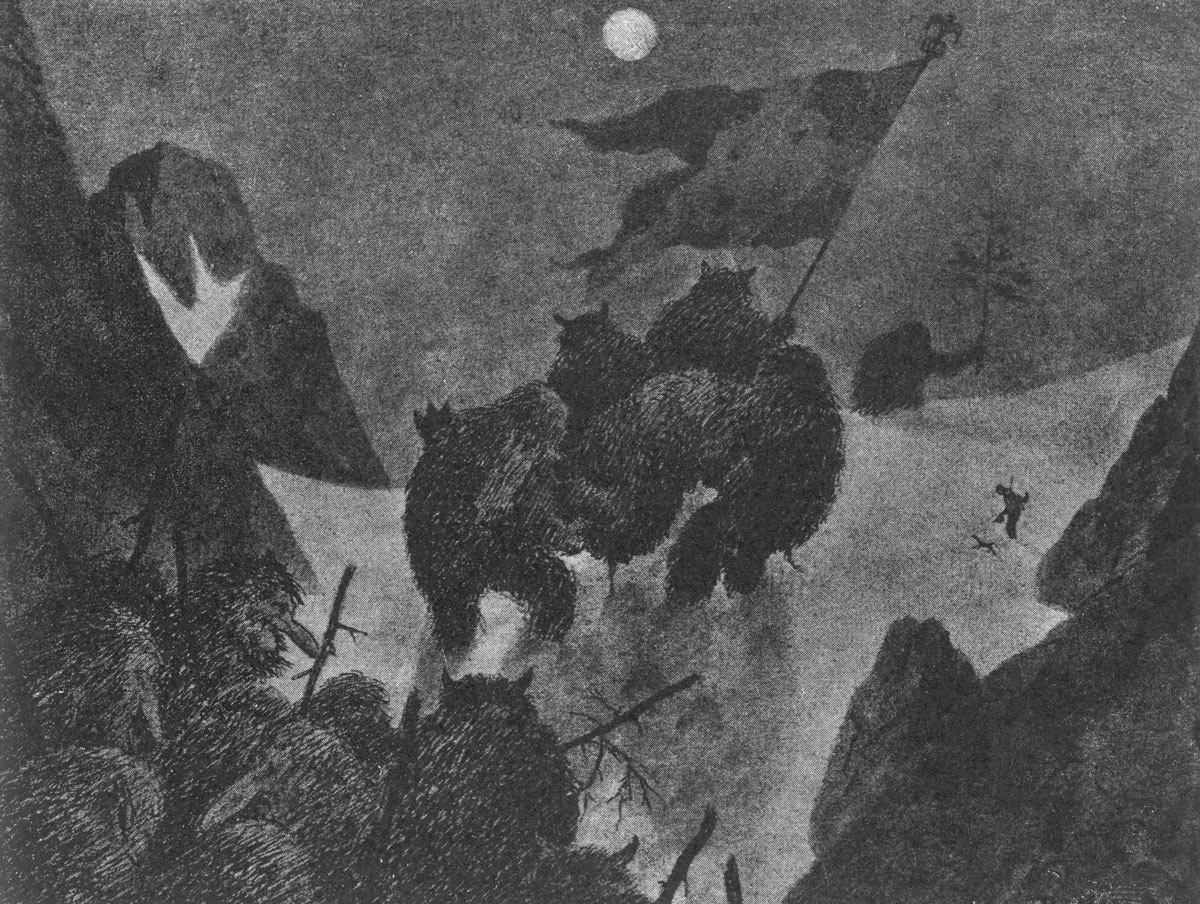A meticulously detailed black-and-white sketch showcases a nocturnal scene set against a backdrop of looming mountains and a prominently positioned moon. The art style, resembling pointillism with its dense array of dots, infuses the image with an ominous, almost ethereal quality. The composition is dominated by tall, furry, wolf-like creatures or Sasquatches descending from the bottom left corner of a canyon or rugged cliffs into a fog-enshrouded area. Among them, one figure at the forefront hefts a large, billowing flag with a dark symbol, while another ahead holds what appears to be a tree branch, possibly as a weapon or staff.

In the middle of the image, these imposing figures seem to be engaged in some form of tension-filled encounter, with the suggestion that they might be carrying a hostage. The ground below is speckled with white, hinting at either snow or mist, contributing further to the eerie ambiance. The shadowy figures are spread across the sketch, with the ones on the right side appearing almost spectral as they move through the fog and darkness. This detailed, monochromatic depiction captures an intense and mysterious scene, rich with emotion and visual drama.